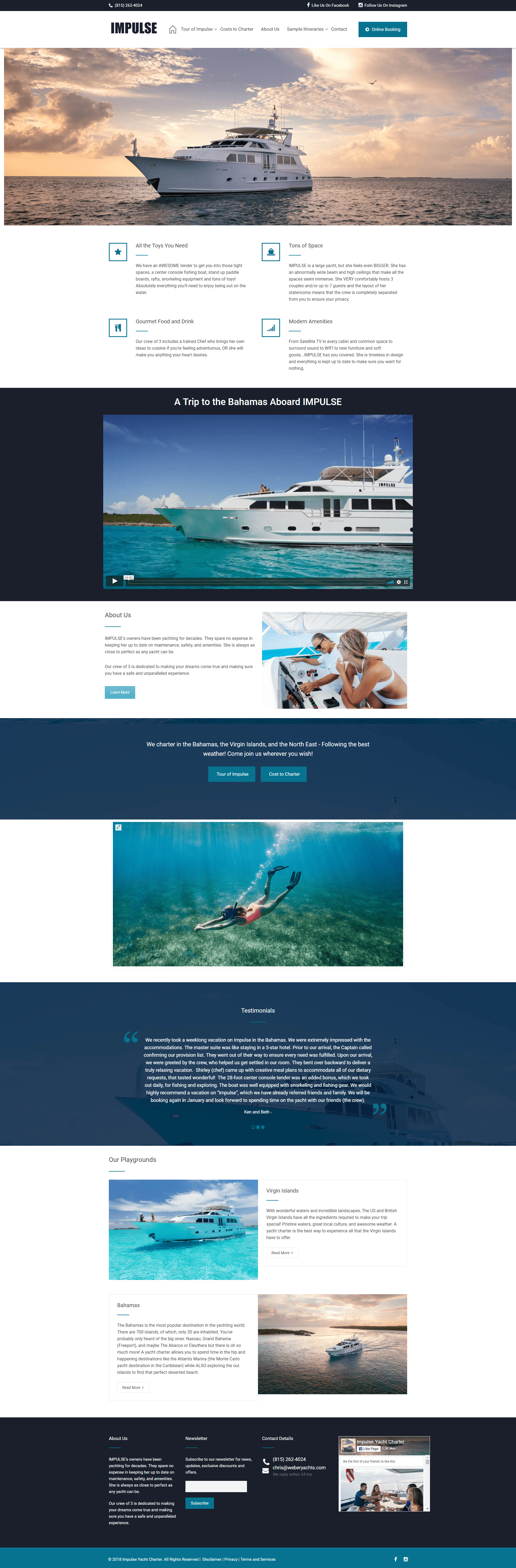Under the "Websites" heading, the webpage features a sleek black bar at the top with a phone number and social media prompts to "Like us on Facebook" and "Follow us on Instagram." Below, a pristine white section showcases the word "Impulse" followed by navigation links: "Tour of the Impulse," "Cost to Charter," "About Us," "Sample Itineraries," and "Contact." A prominent blue button labeled "Online Booking" invites immediate action. The main image captures a stunning yacht named 'Impulse' sitting majestically on the ocean, beneath a vast expanse of fluffy white clouds and bright blue sky. The yacht, impressive in size, promises luxury and adventure. Accompanying text highlights key features: "All the toys you need, tons of space, gourmet food and drink, modern amenities." Below, a captivating video titled "A Trip to the Bahamas aboard the Impulse" plays, showing the yacht navigating through crystal-clear blue waters under a beautiful sky. Two people are seen enjoying the picturesque surroundings. Further down, the section transitions into "About Us," offering more insight into the luxurious yacht experience.